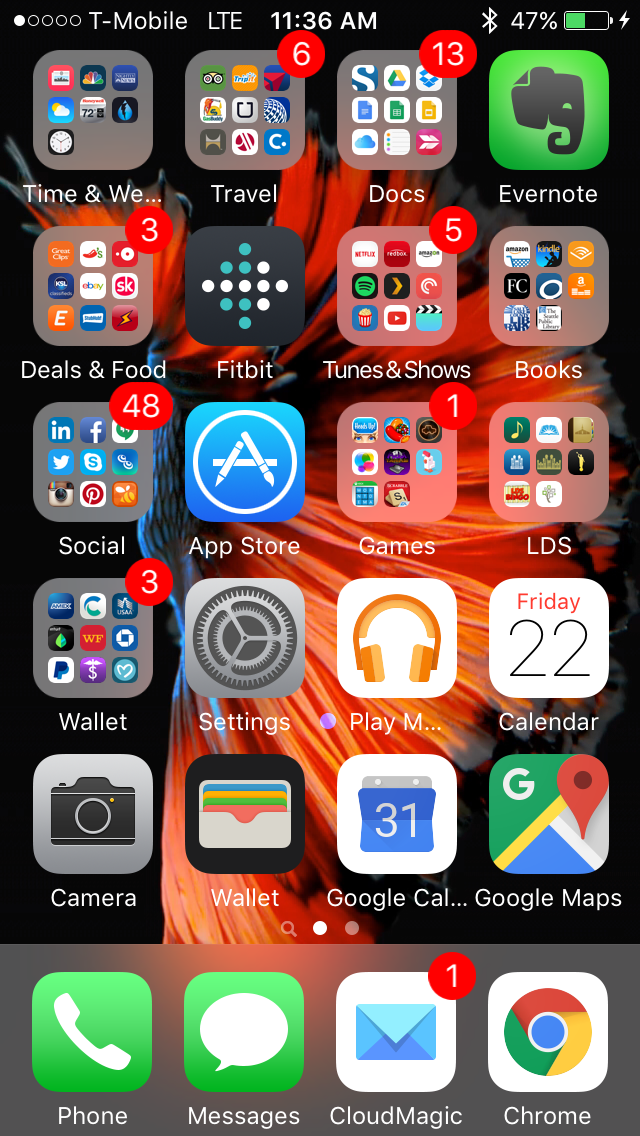This image depicts the home screen of a smartphone, taken from a front view. The device operates on the T-Mobile network, as indicated by the "T-Mobile LTE" label at the top left of the screen. The current time displayed is 11:36 AM, and the battery is showing 47% charge, with an indication that it is currently charging. Bluetooth is enabled on the device.

The bottom section of the screen shows the icons for Phone, Messages, CloudMagic (with a notification badge showing 1 new item), and Chrome. The upper part of the screen features various app groups and individual apps organized in a grid. Notable app folders and icons include:

- Time and Weather
- Travel (showing 6 notifications)
- Docs (showing 13 notifications)
- Evernote
- Deals and Food (showing 3 notifications)
- Fitbit
- Tunes and Shows (showing 5 notifications)
- Books
- Social (showing 48 notifications)
- App Store
- Games (showing 1 notification)
- LDS
- Wallet (showing 3 notifications)
- Settings
- Play Music
- Calendar
- Camera
- Wallet
- Google Calendar
- Google Maps

The background image is predominantly black with vibrant splashes of orange, red, and blue, featuring what appears to be a stylized bird motif.